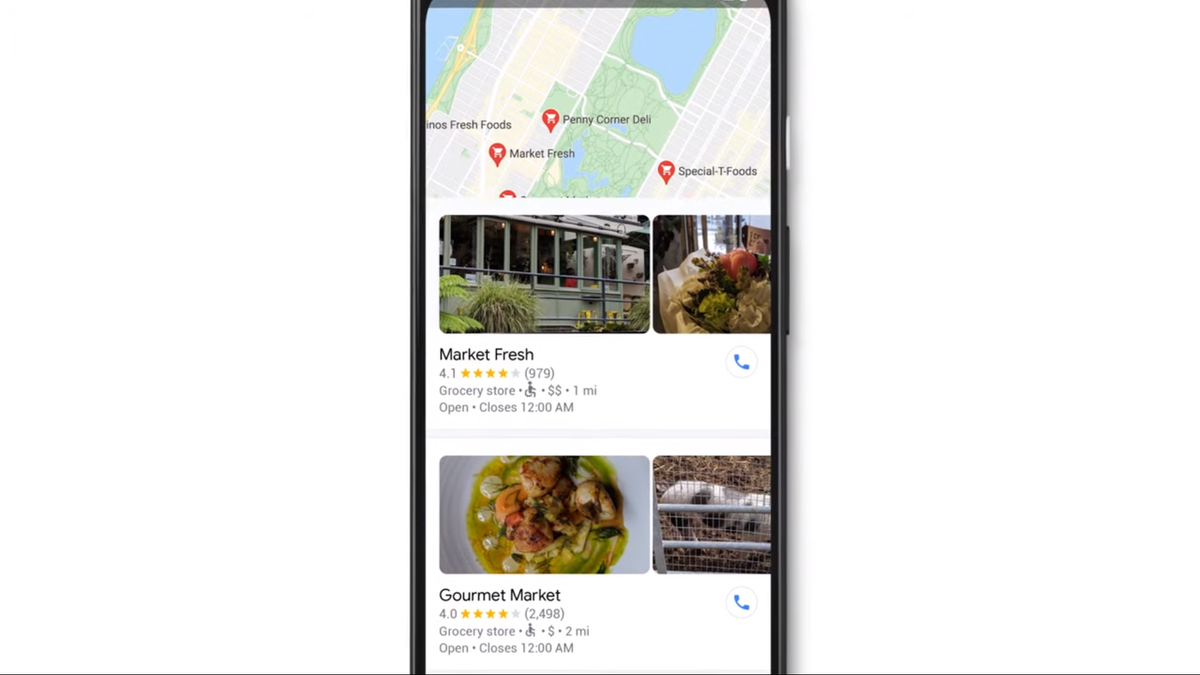This image features a dark-colored cell phone with its top and bottom edges cut off. Displayed prominently on the cell phone screen is a map, showcasing four grocery stores marked with red pins. The map incorporates shades of green and blue in the center and upper left-hand corner, while light gray areas are crisscrossed with numerous roads.

At the top of the map, three pinned grocery stores are clearly labeled: "Penny Corner Deli," "Market Fresh," and "Specialty Foods." Beneath the map, the screen features detailed information about the grocery stores. There are two photos next to the text "Market Fresh," which has a star rating of 4.14 based on 979 reviews, as indicated by the number in parentheses.

Further down, there are two more photos alongside the text "Gourmet Market," which carries a star rating of 4.04. The image captures a real-time view of essential navigational and review data for these grocery stores.